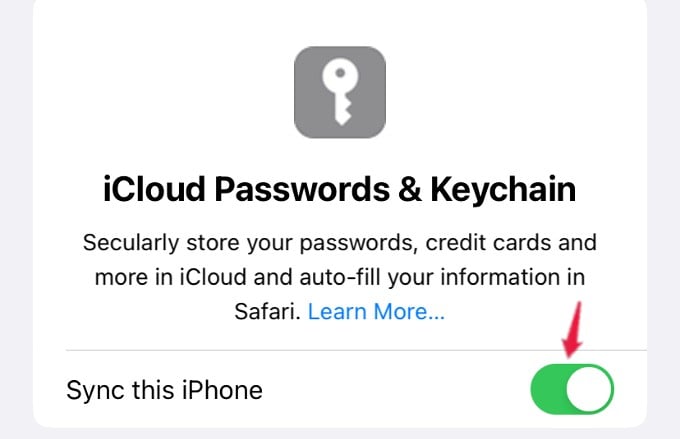The image captures a section of a website dedicated to iCloud Passwords and Keychain. The page header features the title "iCloud Passwords and Keychain" prominently in big, bold, black letters. Below the title, there is an image of a gray square with rounded edges, featuring a white key icon and a gray keyhole that blends seamlessly with the background.

The website layout is framed with light gray borders on the left, right, and bottom sides. Immediately under the main title, the subtitle appears in bold, reading "iCloud Passwords and Keychain" once again. The following text explains the service in clear, large font: "Securely store your passwords, credit cards, and more in iCloud, and autofill your information in Safari."

Further down, there's a "Learn More..." link in blue, inviting users to explore additional details. The website instruction clarity is emphasized by the easy-to-read, large font used throughout.

At the bottom of the page, there is a section labeled "Sync this iPhone," accompanied by a green slider toggle indicating that the sync feature is enabled. A red arrow is directed at the green slider, highlighting the active status of this option. This user-friendly website stands out due to its highly legible text, well-organized layout, and clear instructions, ensuring that users can easily navigate and understand the features offered.